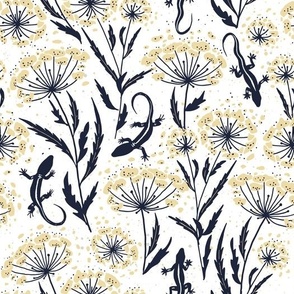The image depicts a square design that closely resembles wallpaper, featuring a cream-colored background adorned with an intricate pattern of flora and fauna. The primary elements include detailed silhouettes of lizards and various flowers, possibly dandelions or Queen Anne's lace. The lizards, numbering at least four, are characterized by their distinctive black silhouettes and white stripes running from their necks to their curled tails, displaying extended fingers on all four feet. Interspersed among these lizards are flowers with long, slender black stems, narrow ridged leaves, and yellow-beige petals. The flowers also exhibit pale peachy-pink puffs and scattered pieces, adding a subtle color variation against the cream backdrop. The overall design has a delicate, illustrative quality, making it suitable for use as wallpaper, fabric, or a vector image background.